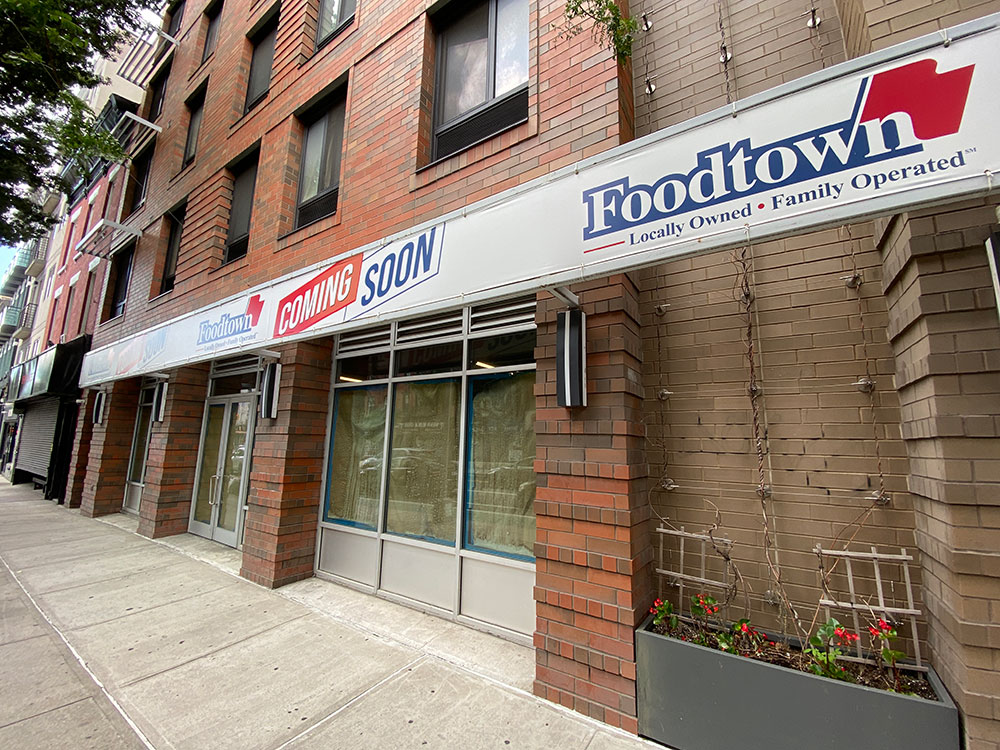The photograph captures a quiet street scene showcasing a brick-layered storefront labeled "Foo Town," a locally owned and operated supermarket in Buffalo. The red-bricked building features three windows and two doors, both of which are covered with blankets or paper, indicating a soft opening. Additionally, a banner on the left side proclaims "Coming Soon." The gray sidewalk in front is spotless and contrasts with a small flower box on the bottom right, housing green plants and red flowers. Adjacent to this structure is a connected brown brick building, likely indicating a mixed-use or residential area, evidenced by balconies and overhanging trees in the vicinity. The street is devoid of people, lending an air of anticipation as the neighborhood awaits the new store's grand opening.